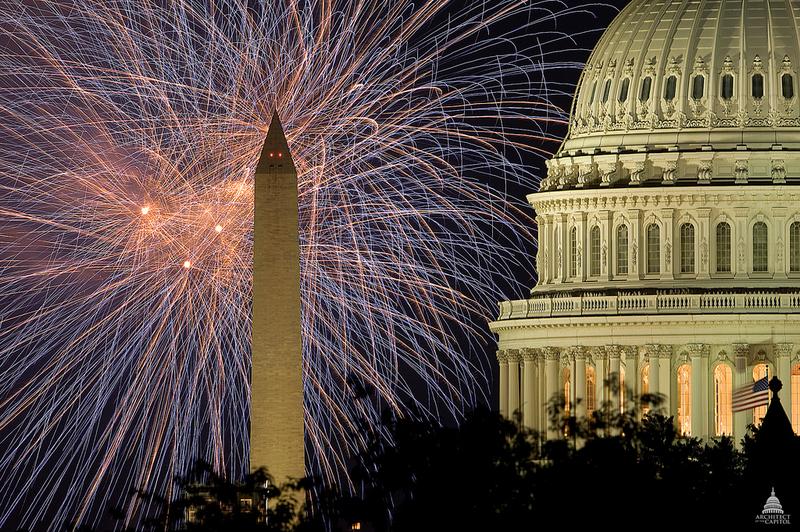The image captures a breathtaking 4th of July fireworks display on the Washington, D.C. National Mall. Dominating the foreground to the right is the iconic Capitol Building, its white dome and elaborate stonework illuminated against the night sky. At its base, dark-shaded trees add contrast to the scene, while the American flag waves proudly in the bottom right corner. To the left, the Washington Monument rises with its signature triangular top and lights at the pinnacle. The background is alive with beautiful, large fireworks exploding in hues of red, blue, and orange, filling the entire left two-thirds of the image. The fireworks' rays radiate across the scene, casting a celebratory glow over this emblematic landscape. The perspective and composition of the elements accurately reflect the grandeur of Independence Day festivities on the National Mall.